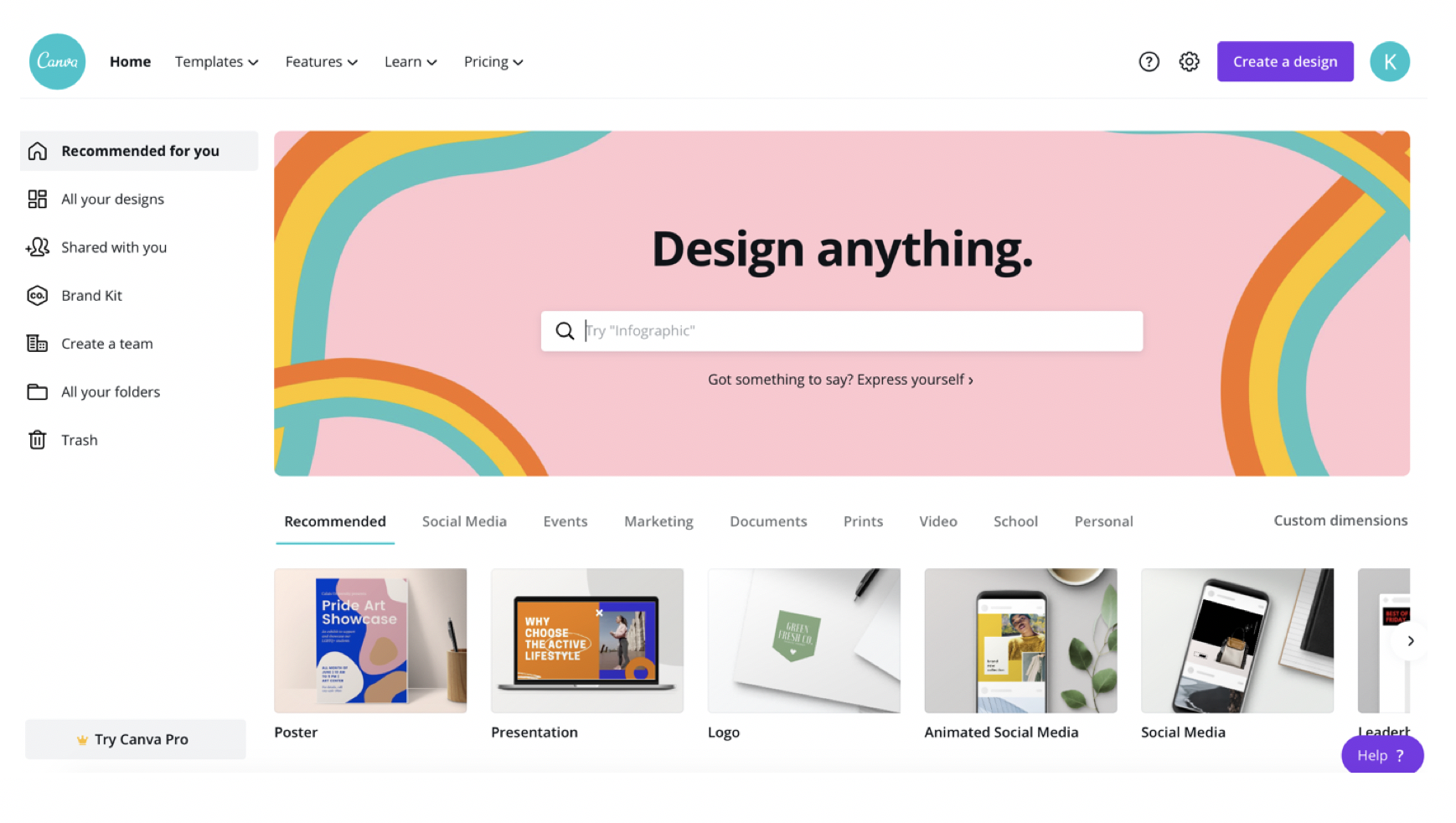In the image, a window of design software is displayed. Dominating the center is a prominent pink box featuring the phrase "Design Anything" in bold black letters. Inside this pink box, to its left and right, are whimsical squiggly lines in teal, yellow, and orange, adding a playful touch. Below this, a white search bar is available, presumably to search contents within the site.

On the left-hand side of the window, there is a vertical menu listing various options such as "Recommended for You," "All Your Designs," and "Shared with You." At the bottom of the interface, tiles offer different design categories to choose from, including options like "Poster," "Presentation," "Logo," "Animated Social Media," and "Social Media."

In the upper right-hand corner, a user appears to be signed in, indicated by the presence of a profile icon with the letter "K" inside it.